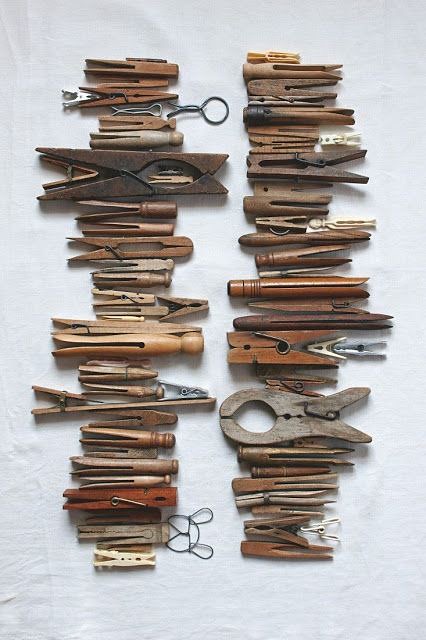The image showcases a collection of antique and modern clothespins, arranged in two rows on a flat white surface. Each row contains approximately 15 pins, displaying a wide range of sizes, shapes, and finishes. The clothespins predominantly exhibit varying shades of brown, from light to dark. Some of the antique pins feature large round knobs for easy gripping, while others use intricate metal mechanisms to provide the required tension. One particular pin stands out due to its enormous size and dark brown color, different from the others. The arrangement captures the evolution of laundry pins, highlighting both their historical and functional variety.